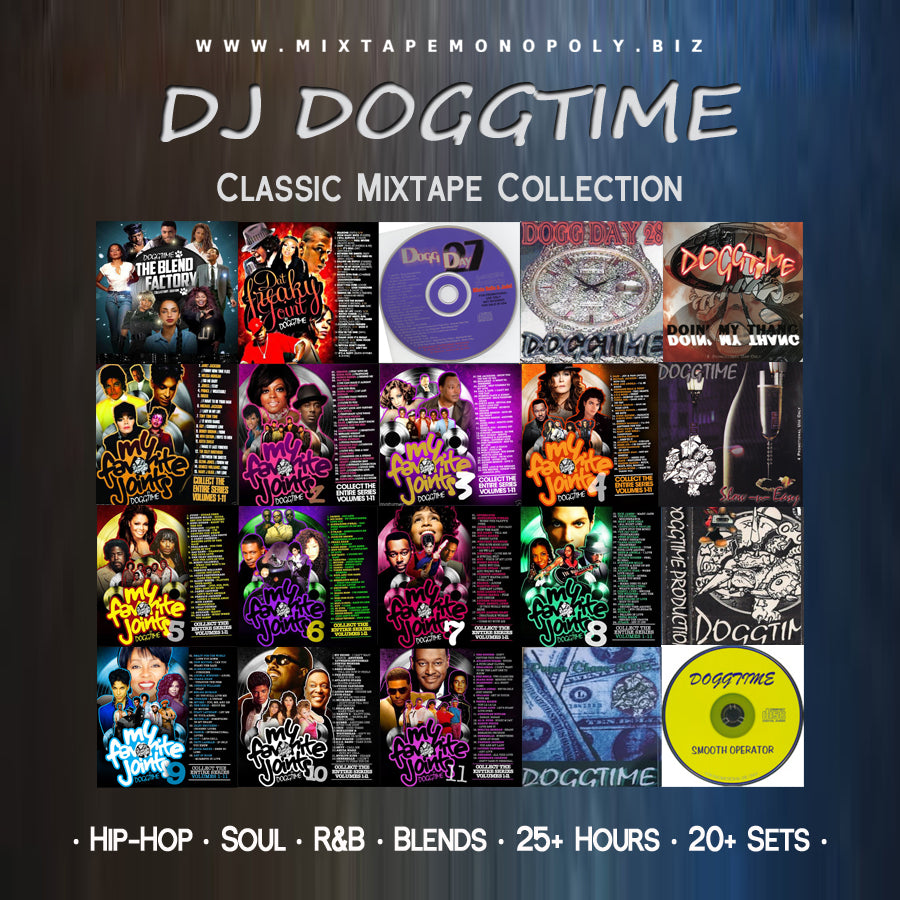The image is an advertisement for the website www.djmixtapemonopoly.biz, featuring DJ Dogtime's Classic Mixtape Collection. The background presents a sleek two-tone silver and bluish-white blend. Prominently displayed at the top in white letters is the website link, followed by "DJ Dogtime" and "Classic Mixtape Collection." The bottom of the image highlights genres including hip-hop, soul, R&B, and blends, boasting over 25 hours of music across 20 plus sets. The central focus is on a grid layout showcasing four rows of five album or mixtape covers, totaling 20 covers. These covers display a range of vibrant colors such as red, black, white, yellow, green, gray, and pink. Among the featured covers, one is yellow, another adorned with money, and a third in purple. Some mixtapes are unopened while others reveal track listings on folded flaps. The collection includes titles like "Factory Blends," volumes 1 through 11, and "DJ Freaky Joint." The overall design is reminiscent of classic CD case art and cassette inlays, capturing the essence of a nostalgic mixtape era with 25 plus hours of hip-hop, soul, and R&B blends.